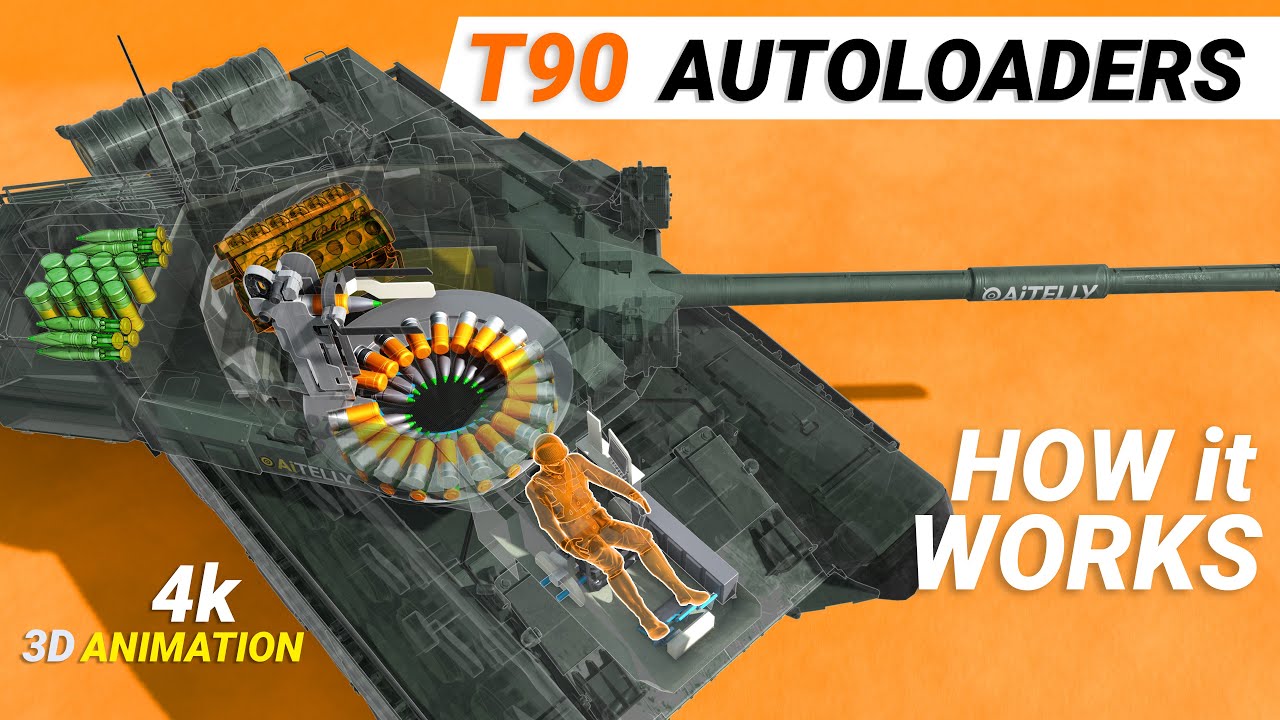The image is a highly detailed, 4K 3D animation, showcasing a computerized x-ray illustration of a T-90 tank. In the upper right-hand corner, bold orange and black text reads "T-90 Autoloaders." The tank itself is depicted in a greenish-gray color against an orange background, with various internal components visible. A silhouette of a person, highlighted in orange, is seated inside the tank, presumably manning it. The tank's ammunition is clearly displayed, with some stored in the center and additional rounds in the back, colored with green tops and yellow bottoms. In the bottom left-hand corner, white and yellow text reads "4K 3D Animation," while the bottom right-hand corner features large white text that states "How it Works." The overall impression suggests this might be part of a video game or educational tool designed to explain the operational mechanics of the tank.